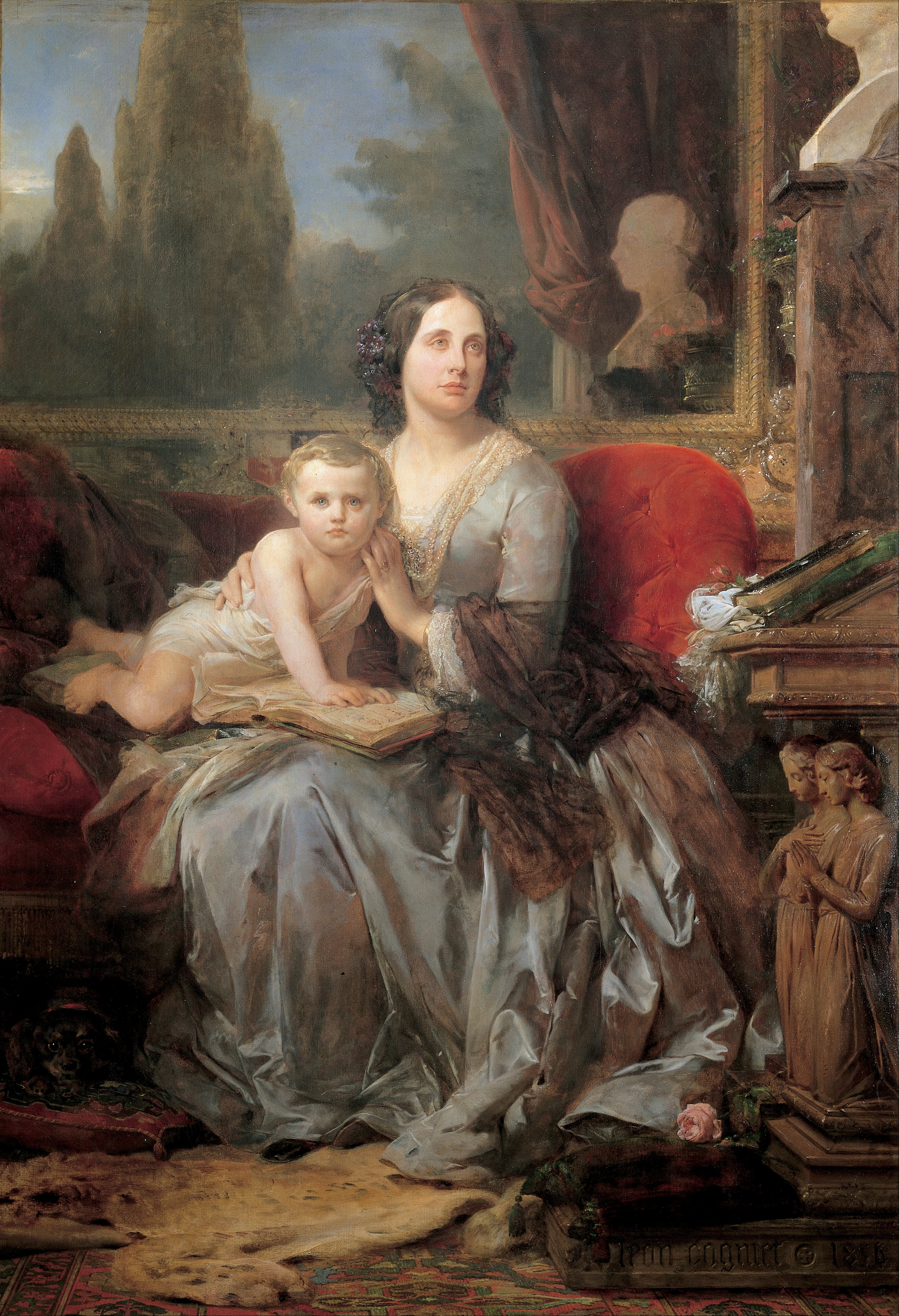This is an elegant 18th- or 19th-century painting depicting a regal woman and her infant child. They are seated on a red tufted sofa. The woman is adorned in a long, flowing gown with shades of green, brown, and gold and a brown scarf draped over her arm. Her dark brown hair, styled with shoulder-length curls, is complemented by a decorative headdress featuring floral elements. Around her neck, she wears beige-colored beads.

The child, who appears to be between one and two years old, is dressed in a white gown reminiscent of classical Greek attire. The child sits in the woman's lap, placing one hand on an open book, their gaze meeting the viewer directly.

The setting is opulent, with a patterned rug beneath them, and to their right, a brown piece of furniture and a statue of two women. The backdrop features a large framed painting of a blue sky and greenery, adding depth and a sense of outdoors. Additionally, there's a hint of a bear rug at their feet and an elaborately designed table with human figure sculptures on its legs. The overall ambiance is one of timeless elegance and maternal grace.